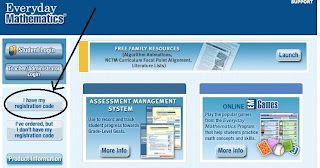In this image, we see a somewhat blurry screenshot of a website with a dark blue header situated in the upper left corner. Inscribed in bold white block letters within this header are the words "Everyday Mathematics, Mathematics." Below this, on the left side, there is a gray box with two items or buttons, though the exact text is unreadable. Further down, there is a black oval outline with the words "Registration Code" inside. Accompanying this text are options in blue: "I have my registration code" and "I've ordered but I don't have my registration code." Underneath these options, there is an action button labeled "Product Information." To the right of this section, there is a long rectangular banner with the word "Launch" prominently displayed on a white button. Below this banner, there are two light blue square boxes, each labeled differently—one reads "Assessment Management System" and the other "Online EM Games."